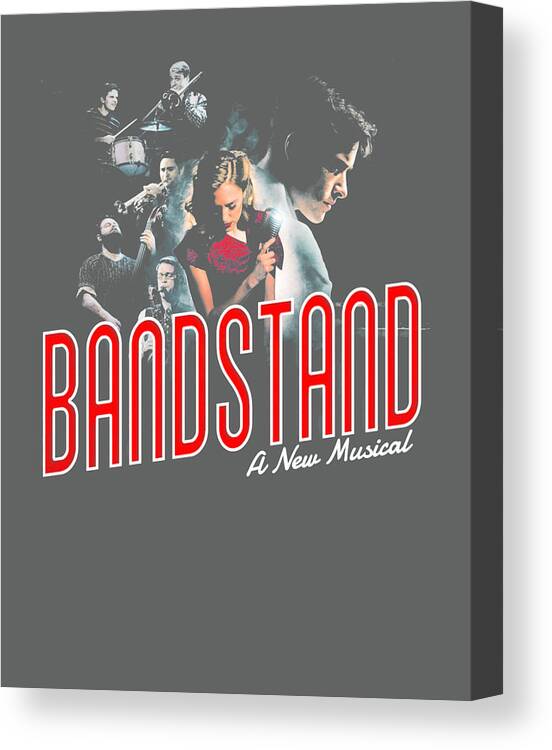The image is a rectangular, gray-colored framed canvas promoting "Bandstand, A New Musical." Dominating the image, the word "BANDSTAND" is prominently displayed in large, red letters with a white outline, positioned centrally. Below, in smaller cursive letters, it reads "A NEW MUSICAL" towards the bottom right. The background features a sepia-toned depiction of a band, including a woman with blonde hair wearing a red shirt, who is passionately singing into a microphone. Surrounding her are various musicians: one playing a trumpet, another on the drums, and another possibly with a cello or violin. The color palette consists of white, red, beige, tan, dark blue, and black, creating a vintage, yet vibrant feel.